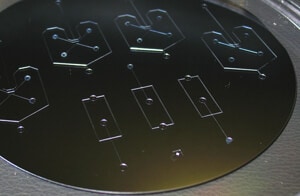The photograph features a close-up of a black metallic circular disc set into a larger gray, hard-surfaced object, likely a piece of machinery. The disc exhibits various intricate engravings and indicators. Notably, along the bottom half of the disc, there are three vertically-oriented rectangular symbols that resemble battery icons, each adorned with three LED-like dots, one positioned centrally and two at the top. The dots on the rectangles at the far left and right are positioned differently from the middle one. Above these rectangles, there are four other engraved symbols, akin to a hinge, each containing four crisscrossing LED-like lights. The disc's surface has patches of light that give it a golden hue in certain areas, adding complexity to its appearance. This detailed arrangement suggests it might be part of an advanced circuit or a battery indicator on industrial equipment.